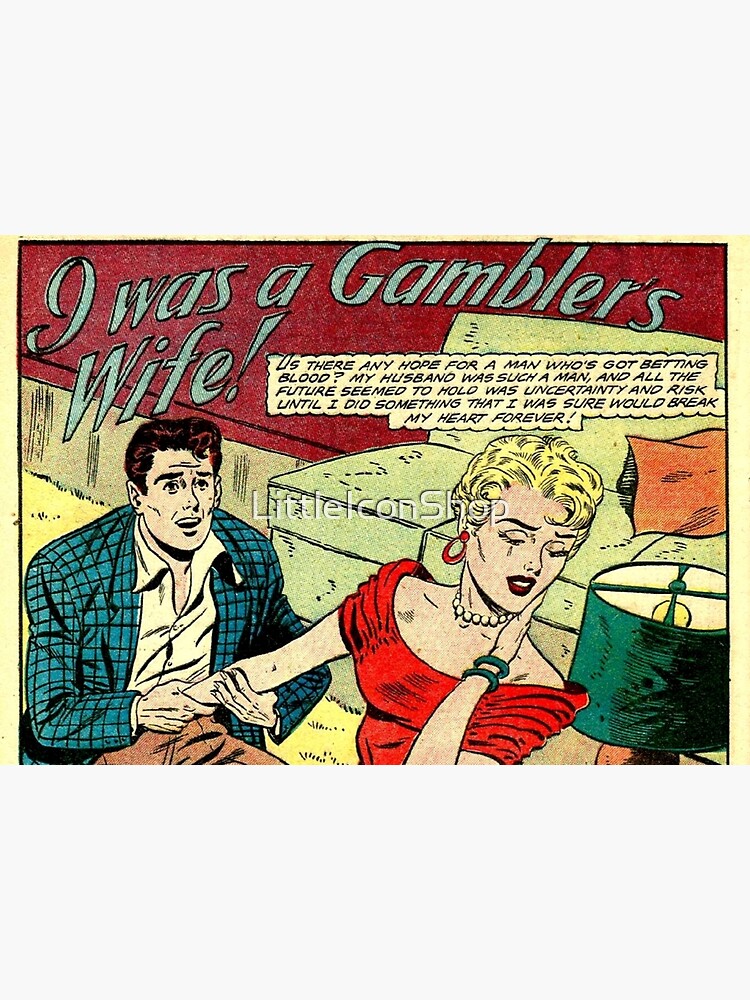This detailed comic book-style illustration captures a dramatic and emotional scene. At the top, the headline in bold gray font reads, "I was a gambler's wife!" Beneath this headline, there's a speech bubble stating, "Is there any hope for a man who's got betting blood? My husband was such a man and all the future seemed to hold was uncertainty and risk until I did something that I was sure would break my heart forever." 

In the panel, a woman in a red off-the-shoulder dress stands crying, a single tear trailing down her right cheek, as she holds her left hand to her face and looks away. She has short, permed blonde hair, is adorned with red hoop earrings and a pearl necklace, and is visibly distressed. Kneeling beside her is a man in a checkered blue jacket with a white dress shirt underneath and brown pants. He has short brown hair and wears a pleading expression as he grasps her arm. 

The setting includes a green sofa in the background and a green lamp positioned at the bottom right corner of the image. Both characters are Caucasian. There's a watermark in the center that reads "Little Icon Shop." The scene vividly portrays a moment of tension and heartbreak, emblematic of classic comic book drama.